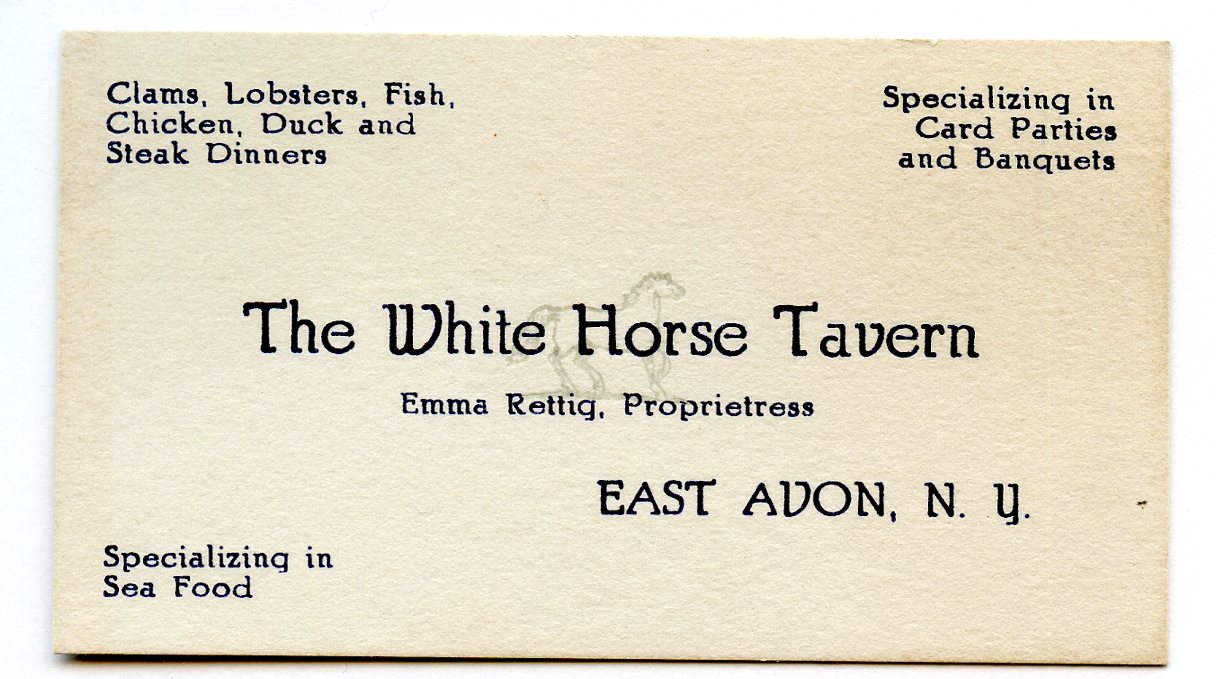The image features a vintage, slightly yellowed business card, likely made of thick, textured off-white cardstock. It is rectangular, longer horizontally than vertically. The card contains multiple lines of black text, detailing the services and identity of the establishment it represents. In the top left corner, it reads, "Clams, Lobsters, Fish, Chicken, Duck, and Steak Dinners" in a small font. The top right corner states, "Specializing in Card Parties and Banquets," also in a small font. The center of the card prominently displays "The White Horse Tavern," beneath which "Emma Rettig Proprietess" is written, followed by "East Avon, NY." A semi-transparent, faint grey outline of a horse serves as a background watermark behind the central text. In the bottom left corner, the text indicates, "Specializing in Seafood." The overall aesthetic suggests an older, somewhat aged business card.